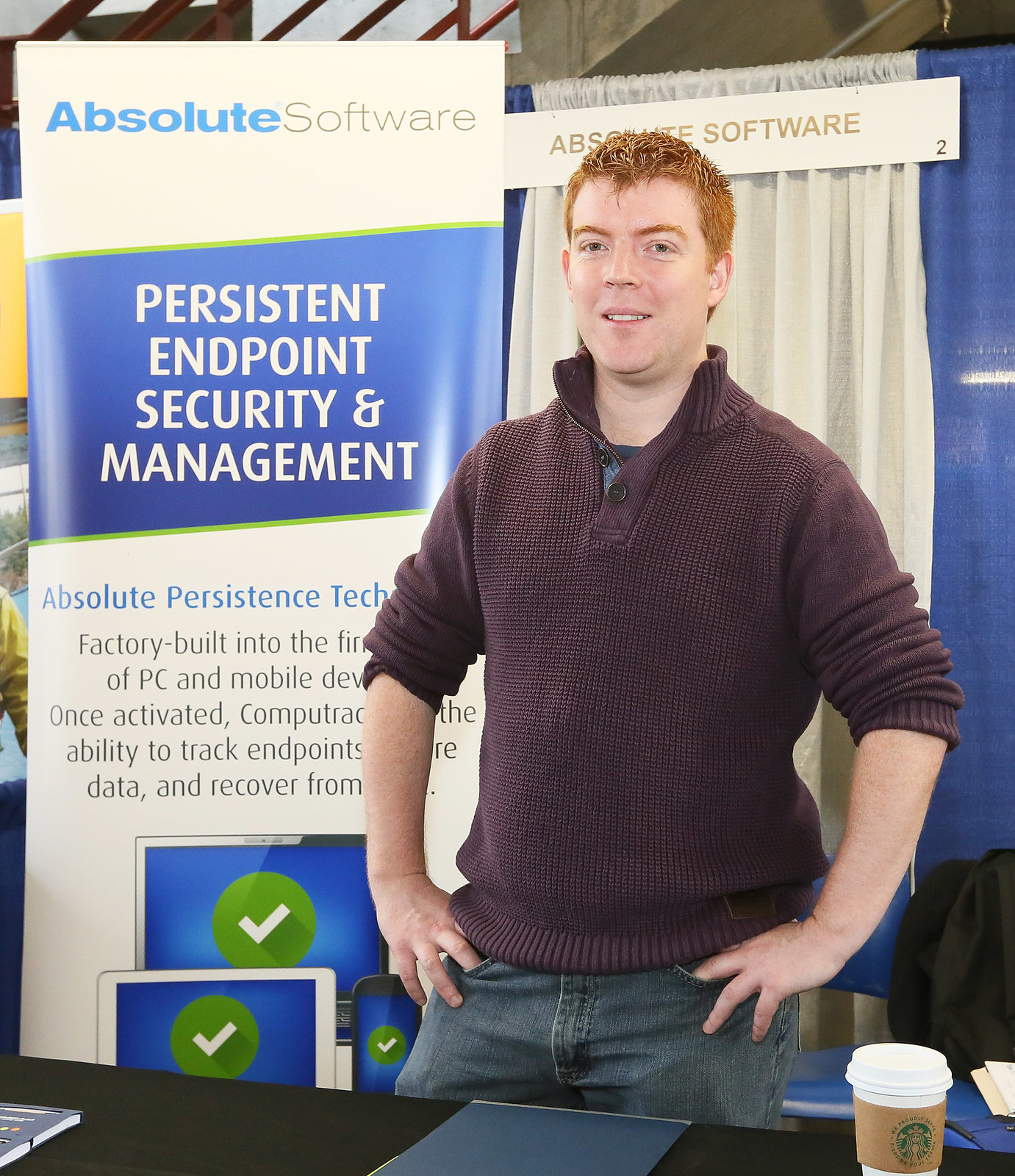This image captures a man with short, heavily gelled red hair and matching red eyebrows, posing with both hands on his hips and giving a somewhat uncomfortable smile. He is dressed in a collared purple sweater with rolled-up long sleeves and blue jeans, though only the tops of his jeans are visible as he stands behind a black table. On the table in front of him, there's a white Starbucks cup with a sleeve, positioned to his right, and a blue piece of paper below him. A partially visible book lies on the table as well. 

Behind him, a banner reading "Absolute Software" in white letters on a blue background is displayed. This banner also features the words "Persistent Endpoint Security and Management" outlined in green, accompanied by clipart images resembling a laptop, a phone, and perhaps an iPad screen. Additionally, another white sign with gold lettering that says "Absolute Software" along with the number two is partially visible near his head. The background also shows the chair back, suggesting seating is available, and the faint presence of another person’s arm is seen to the left, between the banner and some empty space.